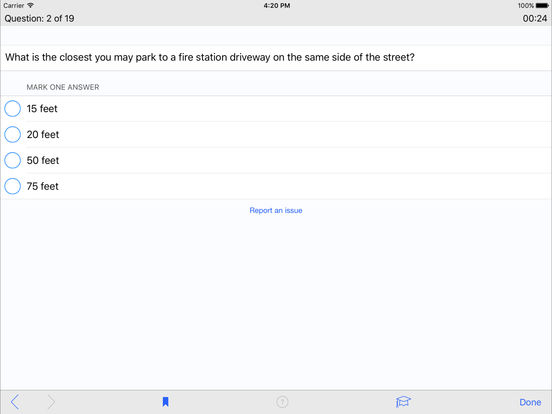This screenshot captures a segment of an online quiz, specifically focusing on traffic regulations. At the top, it indicates the quiz's progression, labeled "Question 2 of 19." The question posed in this section reads, "What is the closest you may park to a fire station driveway on the same side of the street?" Participants are instructed to select one answer from the provided choices. The available responses include 15 feet, 20 feet, 50 feet, and 75 feet. Positioned beneath the options is a clickable text in blue stating, "Report an issue." The layout suggests a user-friendly interface, guiding users through the quiz with clarity.